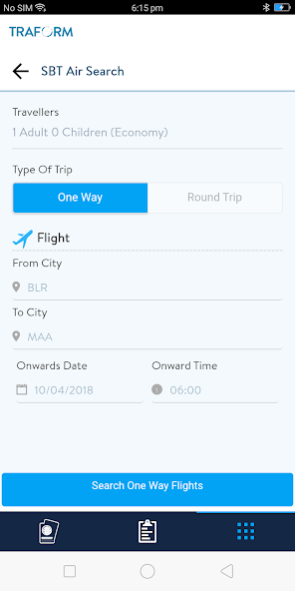The screenshot displays a travel booking interface on a user's phone. At the top of the screen, a thin black banner indicates the time as 6:15 p.m. on the left, while on the right, a battery icon shows half charge with a white thunderbolt. The status "No SIM" is also visible on the left side of this banner.

Below this, in bold bright blue capital letters, the header reads "TRAFORM." Underneath it, on a light bluish-green background, the text "TRAVELERS" is displayed in gray. This section details the journey specifics: "One Adult, Zero Children, Economy (in parentheses)," followed by a gray text header "TYPE OF TRIP."

The interface offers two options for trip type: a bright blue button labeled "ONE WAY" in white, and a white button labeled "ROUND TRIP" in gray.

Further down, a bright blue airplane icon precedes the word "FLIGHT" in gray. The travel details include departure city "FROM CITY: BLR" and destination "TO CITY: MAA." The dates and times for the journey are specified as "ONWARDS DATE: 10-4-2018" and "ONWARD TIME: 6:00."

At the bottom, a sky-blue banner spans the screen with the CTA "SEARCH ONE WAY FLIGHTS" in white text. Below this, a navy-blue banner with various icons is visible. The screen's bottom-most section features a light gray banner housing navigation buttons: "HOME," "BACK," and "REFRESH."

This interface layout blends clear visual indicators and textual information to facilitate a seamless travel booking experience.